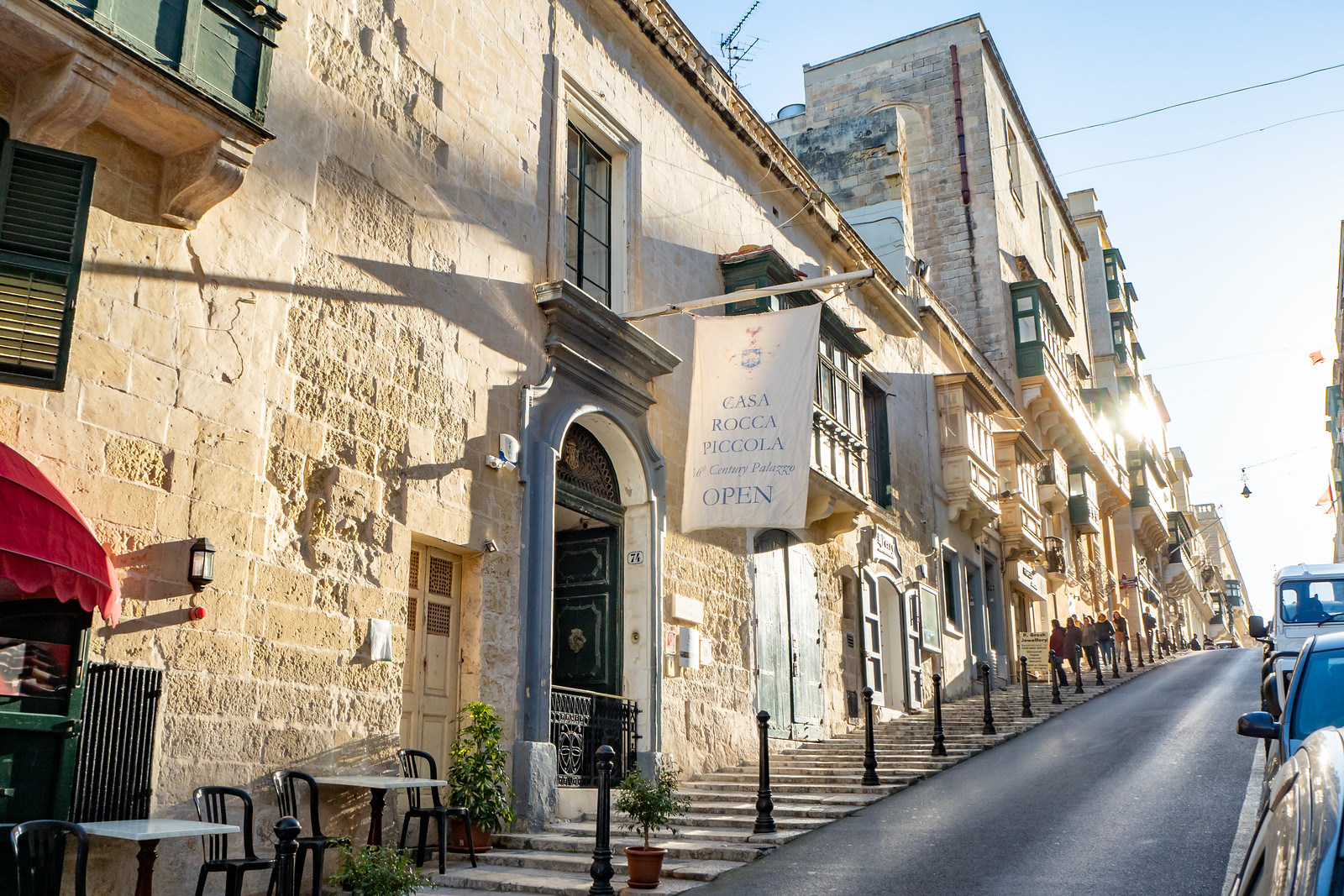This photograph captures a vibrant street scene featuring a central gray road flanked by contrasting elements. On the left side, the sidewalk transforms into white steps due to the sloped, uneven terrain. These steps are bordered by black metal banisters, guiding pedestrians as they descend. Adjacent to the street are old, stone buildings with green-colored walls, reminiscent of European architecture, dating back to the 16th century. One building has a white flag with blue text reading, "Casa Roca Piccola 16th century palazzo open." This particular building also features outdoor seating with tables and chairs. Amidst the clear blue sky, people are seen walking down the steps, possibly shopping or touring the historic area. On the right side of the road, there are vehicles moving along, contributing to the dynamic atmosphere of the scene.